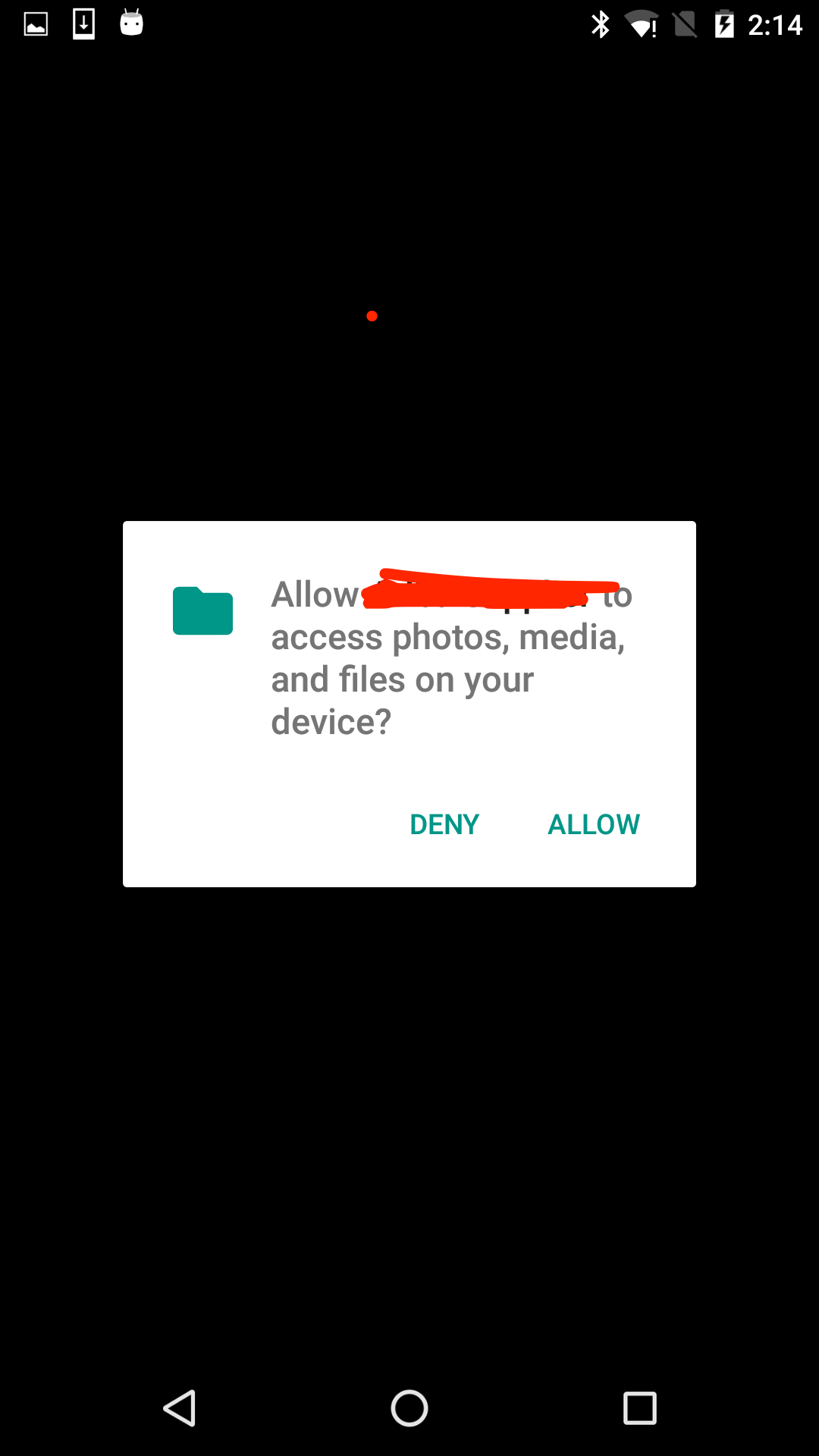This image appears to be a screenshot taken from a cell phone, displaying a permission request pop-up. The background of the image is entirely black, creating a stark contrast with the white rectangular pop-up in the center. The pop-up features a message that has been partially obscured by a red scribble, making it impossible to read certain portions of the text. The visible part of the message reads: "Allow [blank] to access photos, media, and files on your device."

In the top-left corner of the white rectangle, there is an icon resembling a file folder. At the bottom of this pop-up, there are two clickable options: "Deny" on the left and "Allow" on the right.

Above the pop-up, the phone's status bar is visible. In the top-right corner, the time is displayed as "2:14," next to a battery life icon, and three additional, tiny icons. In the top-left corner of the status bar, there are three more tiny icons. In the middle of the otherwise black upper space, a single dot is present, seemingly a subtle detail left by whoever scribbled out the personal information. 

At the bottom of the screenshot, against the black background, are three navigation icons common to many Android devices: a triangle (back button), a circle (home button), and a square (recent apps button), all in white.